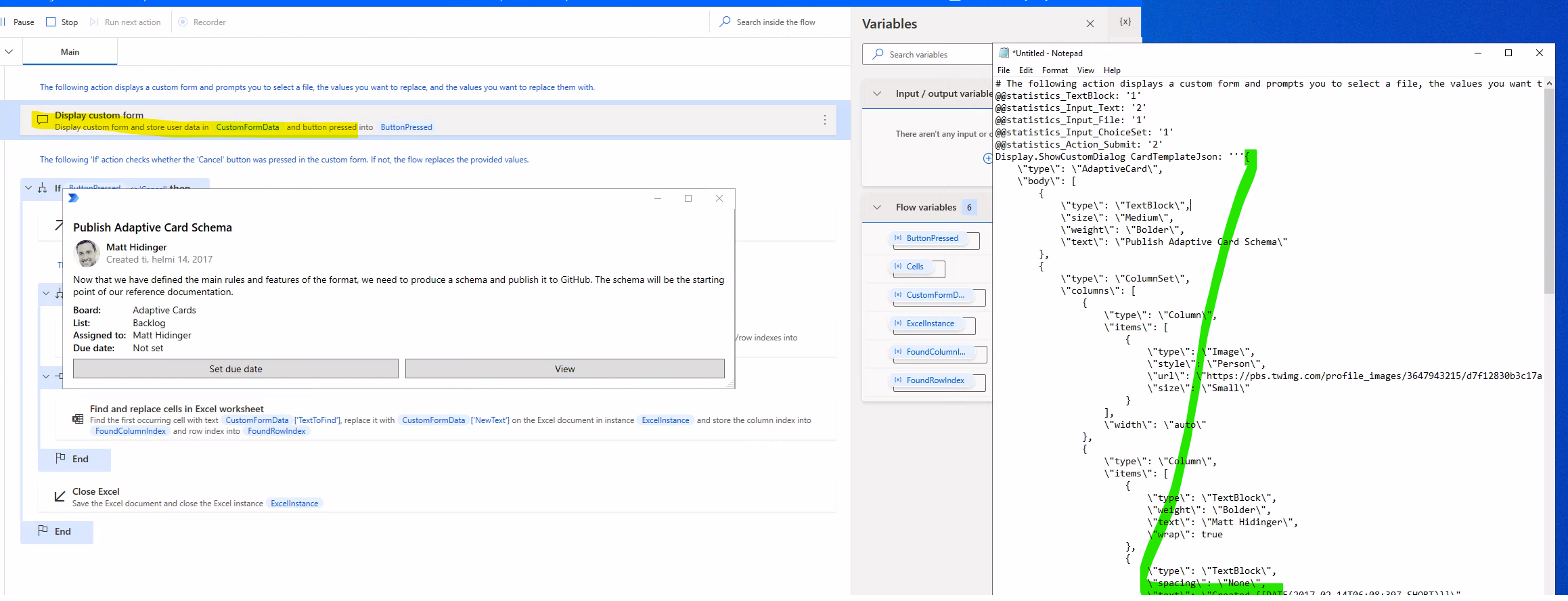The image depicts a slightly blurry screenshot of a website, likely showcasing a coding environment. In the background, there are two main sections: the foremost screen displaying a box with "Untitled - Notepad" near the top right, filled with lines of code, including a peculiar green-highlighted 'l'. The secondary screen behind it features a bar at the top labeled "variables" in a gray box and a larger white-framed section. Within this section, a smaller box contains the words "Publish Adaptive Card Schema" and instructions for "Set the date or view." All of these elements are displayed against a blue background, suggesting a multi-window layout on a computer desktop. The overall screenshot is somewhat difficult to decipher due to its blurriness.